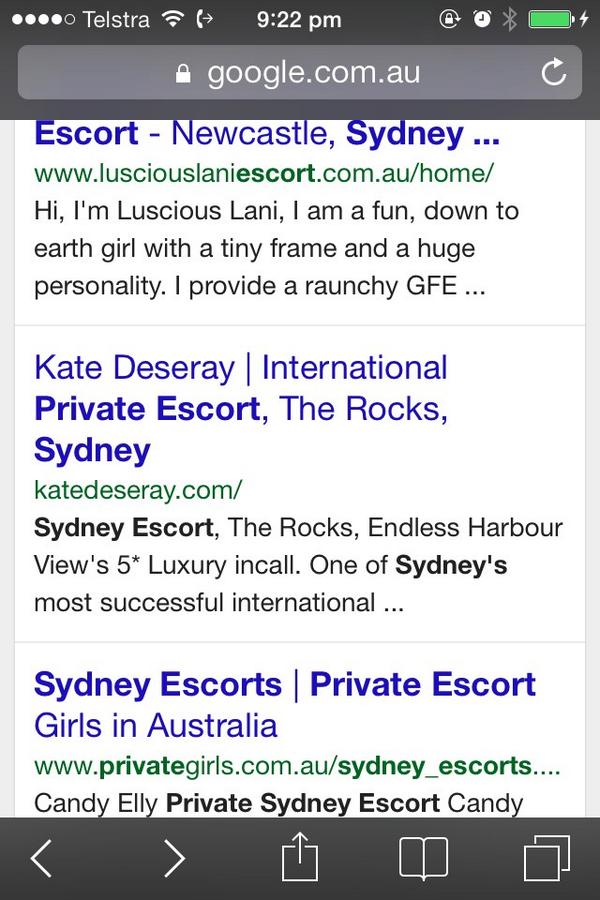This image is a screenshot taken from a mobile device, capturing a web browser interface. At the top, a dark grey header displays various white icons indicating WiFi connection, network status, time, Bluetooth connection, and battery life. Directly below this header lies the web address bar with a light grey background, containing the text "google.com.au." 

Beneath the address bar, the screen shows the first three search results for escort services in Sydney, Australia. Each result features a blue hyperlink, followed by a green web address and a brief description in black text. 

At the bottom of the screen, the footer includes several navigational icons such as forward and backward arrows, along with options to copy and paste text. The interface elements collectively create a clear snapshot of an active search session on a mobile web browser.